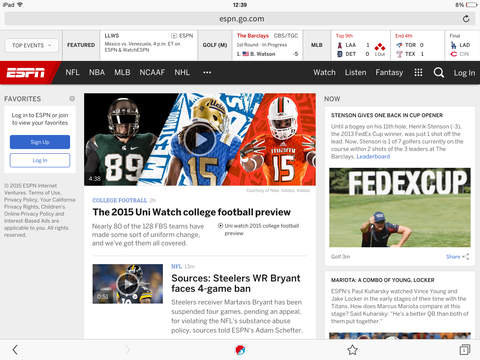This screenshot appears to be taken from an iPad, as indicated by the gray status bar at the top displaying the black font text: "iPad," with a full Wi-Fi signal icon, the time "12:36 PM," and the battery level at a critical 8%. Below the status bar, the Safari browser is open, showing a web page from "ESPN.go.com." 

At the top of the webpage, a navigation bar is visible, offering links to "Top Events" and "Featured." Below this navigation bar, there are several article titles related to various sports, including "Golf," "MLB," and "The Barclays." While there appears to be game scores in the upper right corner of this section, they are too small to read clearly.

Further down, there is a black horizontal bar with a small red square in the upper left corner featuring the white ESPN logo. Following the logo, the black bar displays, in white font, the sections: "NFL," "NBA," "MLB," "NCAA," "FNH," "NHL," and additional options symbolized by an ellipsis (...). To the right of these sections, the bar includes a magnifying glass icon, indicating a search function, and the text "Log In."

At the bottom of the screenshot, there is a gray vertical rectangle prompting users to log in or sign up. The text within this rectangle reads, “Favorites: Log into ESPN or join to view your favorites. Sign up or log in.”